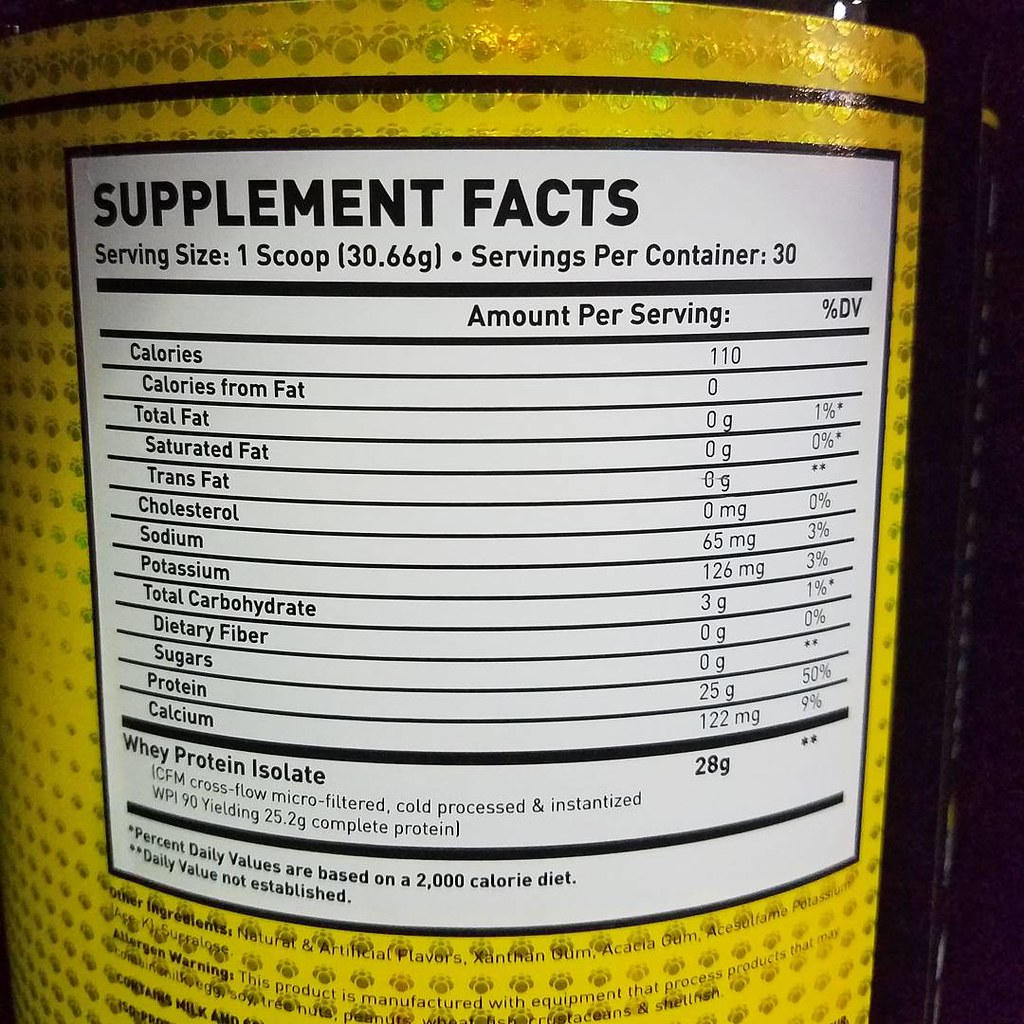This detailed photograph captures a close-up view of the nutritional facts label on a round, bright yellow container of whey protein isolate. The yellow tub is adorned with a holographic gold circular pattern that spans its background, save for where the large white label dominates the foreground. At the top of the label, bold black text reads "Supplement Facts." Detailed information follows, specifying a serving size of one scoop, equating to 30.66 grams, with the tub containing 30 servings per container. The label lists the caloric content as 110 calories, with zero calories from fat, and breaks down the macronutrients and micronutrients as follows: 

- Total Fat: 0g 
- Saturated Fat: 0g 
- Trans Fat: 0g 
- Cholesterol: 0mg 
- Sodium: 65mg (3% DV)
- Potassium: 126mg (3% DV)
- Total Carbohydrate: 3g (1% DV)
- Dietary Fiber: 0g
- Sugars: 0g
- Protein: 25g (50% DV)
- Calcium: 122mg (9% DV)

Additional information indicates the presence of Whey Protein Isolate, 28g, with specifics on its processing methods—Microfiltered, Cold Processed, and Instantized—yielding 25.2g of protein. There is also a note that Percent Daily Values are based on a 2000 calorie diet. Further down the label, in black text, are details on other ingredients and allergen information. The top of the picture shows a black line, hinting at the tub's opening mechanism through a perforation.